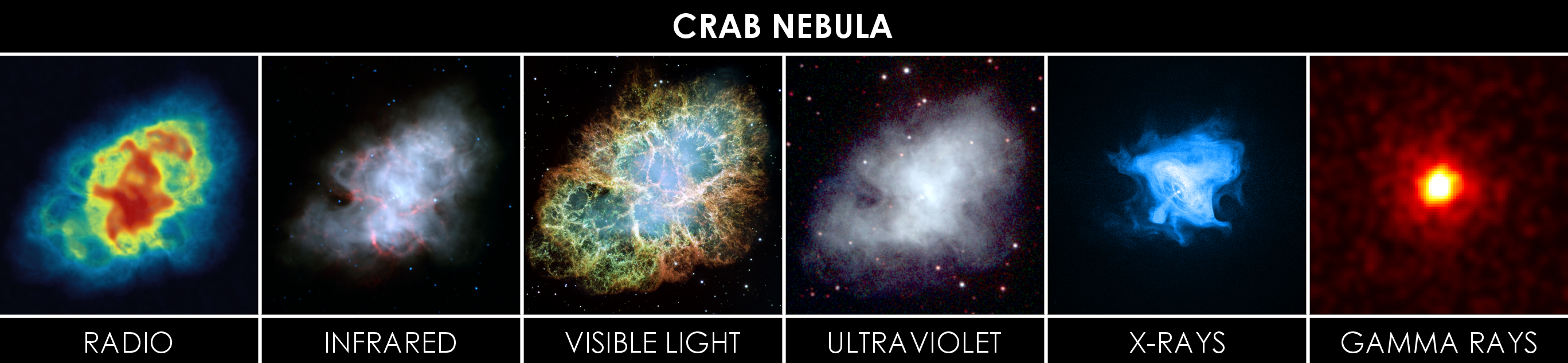This horizontally oriented composite image from a scientific study features six different representations of the Crab Nebula, each captured in a distinct wavelength of the electromagnetic spectrum and arranged against a black background. The images are labeled with their respective wavelengths: 

1. **Radio Waves**: Depicted in colors of blue on the exterior with red on the interior.
2. **Infrared**: A blend of light lavender and orange.
3. **Visible Light**: Bright green, intertwined with yellow highlights.
4. **Ultraviolet**: Resembles a white puff of smoke, indicative of a cloud-like appearance.
5. **X-rays**: Electric blue with a distinctly bright white center.
6. **Gamma Rays**: Displays a hot yellow core transitioning to red on the edges.

Each image captures a unique aspect of the Crab Nebula, providing a comprehensive view across multiple wavelengths, revealing the dynamic nature of this celestial object. With "Crab Nebula" inscribed at the top, this layout is reminiscent of a film strip or textbook excerpt, effectively illustrating the diverse emissions from the nebula.